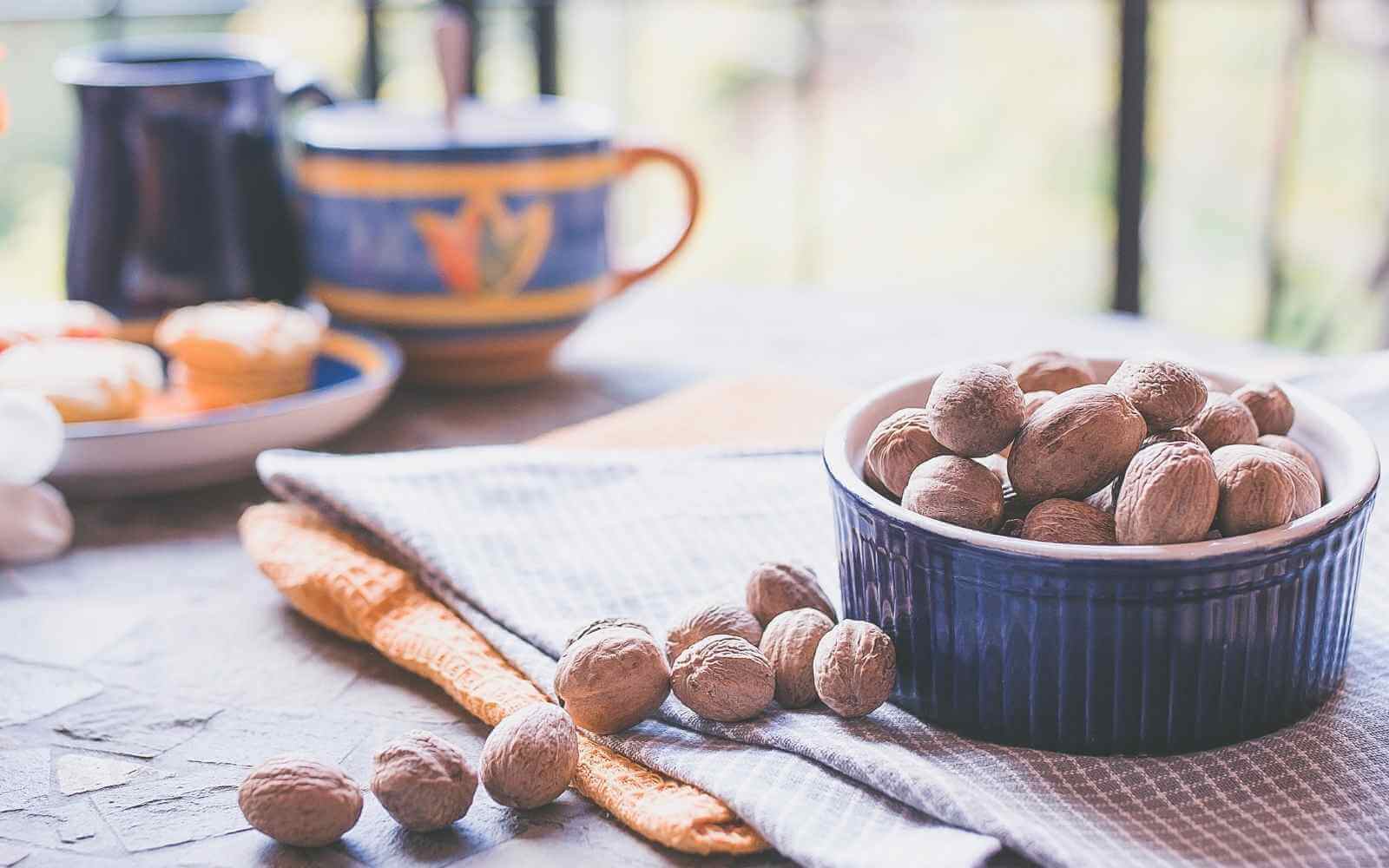In this brightly lit kitchen setting, an inviting scene is captured featuring a blue ceramic bowl with a white interior brimming with light brown nuts, potentially walnuts or chestnuts, still in their shells. The bowl is placed on a folded white and blue checkered napkin atop a yellow gold waffle-knit towel. Ten of these nuts lie scattered to the left of the bowl on a textured brown countertop. To the top left of the composition, a dark blue ceramic jug stands next to a blurred blue and yellow ceramic cream container and a small plate adorned with what appears to be muffins or Danish pastries. The image, bathed in sunlight suggestive of proximity to a window, conveys a homely, cozy atmosphere, with the nuts and the bowl in sharp focus against a softly blurred background.